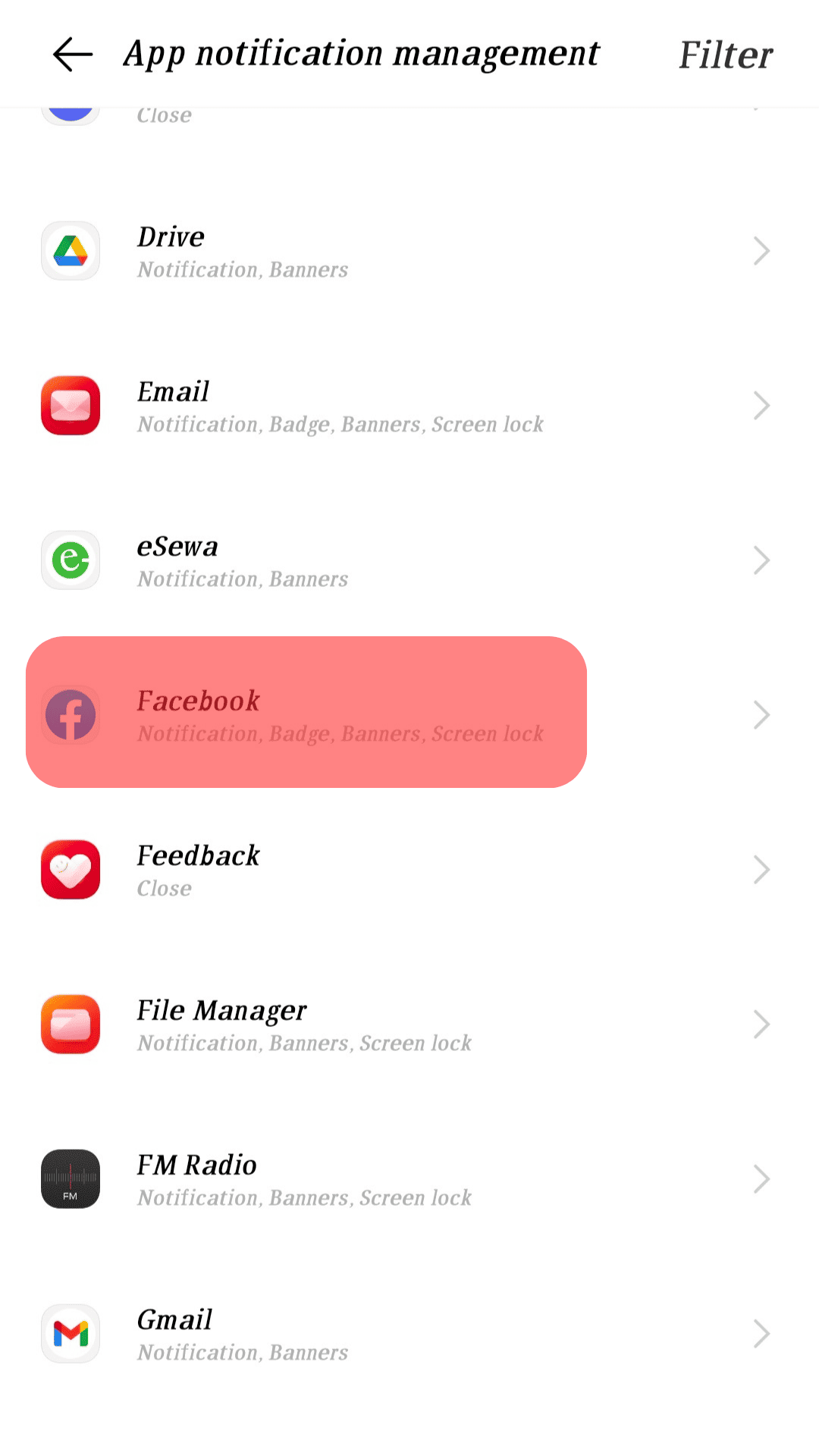**App Notification Management**

The image shows various elements related to app notification settings. At the top right, there is black italicized text in the Georgia font that acts as a header, reading "App Notification Management."

On the far left, there is italicized text that also appears to be in the Georgia font, which says "Filter." Proceeding to the right, there is a black arrow pointing left, leading into a list of applications.

1. **First Application (Partially Visible)**
   - A purple end of a circle is visible with the text "Close" beside it.

2. **Drive**
   - Icon: The Google Drive symbol towards the left.
   - Text: "Drive"
   - Description: Below the title, in gray italicized lettering, it reads "Notification, Banners" with a gray arrowhead pointing right.

3. **Email**
   - Icon: A dark red background rounded square with a transparent envelope in the middle.
   - Text: "Email" in black bold italicized lettering.
   - Description: Below the title, in gray italicized font, it reads "Notification, Badge, Banners, Screen Lock" with a gray arrowhead pointing right.

4. **EWA**
   - Icon: A white background with a gray border, containing a green filled-in circle with a slanted white "e" resembling Times New Roman font.
   - Text: "eSewa" (with "lowercase e, capital S, and lowercase ewa" in black bold italicized lettering).
   - Description: Below the title, in smaller gray italicized lettering, it reads "Notification, Banners" with a gray arrowhead pointing right.

5. **Facebook (Highlighted in Red)**
   - Icon: A circular icon with the Facebook logo.
   - Text: "Facebook" in bold italicized lettering.
   - Description: Below the title, in smaller italicized font, it reads "Notification, Badge, Banners, Screen Lock."